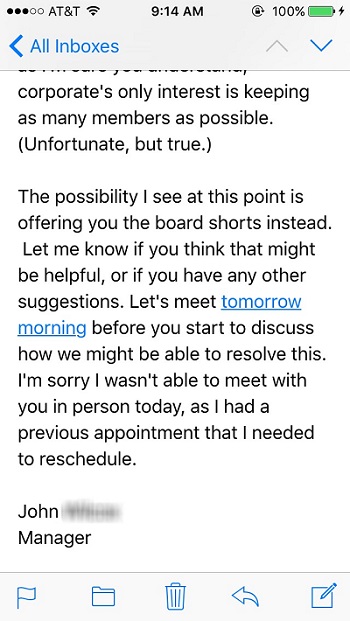Here is a cleaned-up and detailed caption for the described image:

---

The image captures the screen of a tablet or smartphone, powered by AT&T, displaying an email interface labeled "All Inboxes." At the top, a blue left-arrow icon is visible, indicating the option to navigate back. Below this, the email content is partially visible, having been scrolled down to the middle of a paragraph.

The visible portion of the email begins mid-sentence, stating, "Corporate's only interest is keeping as many members as possible. Unfortunate but true. The possibility I see at this point is offering you the board shorts instead. Let me know if you think that might be helpful or if you have any other suggestions."

A key part of the email, highlighted in blue and underlined for emphasis, reads, "Let's meet tomorrow morning before you start to discuss how we might be able to resolve this."

The email continues with an apology for not being able to meet in person due to a prior appointment, concluding with, "I'm sorry I wasn't able to meet with you in person today as I had a previous appointment that I needed to reschedule."

The email is signed off by "John," with the last name obscured, and includes his title, "Manager."

Overall, the tone of the message appears sincere and professional, addressing an issue and proposing a face-to-face meeting to find a viable solution.

---

This detailed caption clarifies the context and content of the email displayed on the screen.